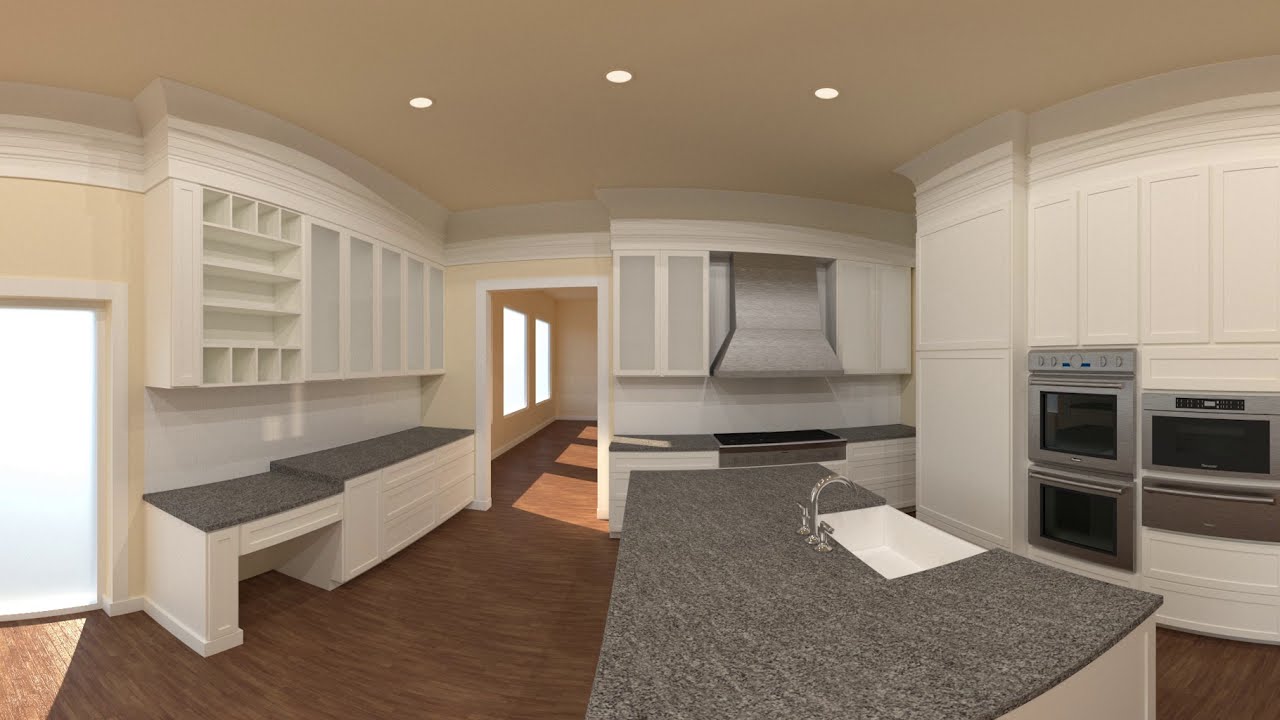The image depicts an upscale, modern kitchen, likely an AI-generated or real estate photo emphasizing its pristine and vacant state. At the center of the kitchen is a sleek, thin island topped with gray granite, contrasting a white base visible on the right side. The right side of the kitchen features built-in chrome stove and microwave units, adorned with tinted glass doors and flanked by white cabinets against a matching white wall. Shelving and additional granite countertops, some with varying heights, line the left side. A doorway in the left wall opens into an adjacent room illuminated by natural light streaming through two windows. The floor boasts dark brown hardwood planks, exuding a warm, rich tone. The ceiling above is light yellow with three recessed circular lights. Additional features include ample cupboard space, a designated area for a refrigerator, sliding doors, and a small nook for shoes near the entrance, emphasizing the kitchen's functionality and elegance.